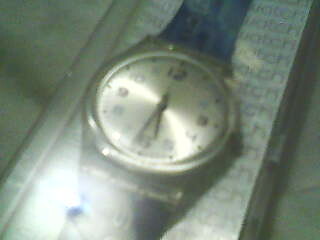A slightly blurred photograph captures a classic timepiece resting on its thin display box, seemingly taken through a glass display that adds a reflective sheen to the image. The watch, composed of both silver and gold metal, features a round silver face adorned with numerals 1 through 12, precisely indicating the time at 5:31. Attached to the watch is a dark wristband, contrasting elegantly with the metallic tones of the timepiece. The box, which the watch sits upon, displays a visible hinge on one side and is placed atop a gray surface, adding a subdued yet sophisticated backdrop to the overall scene.